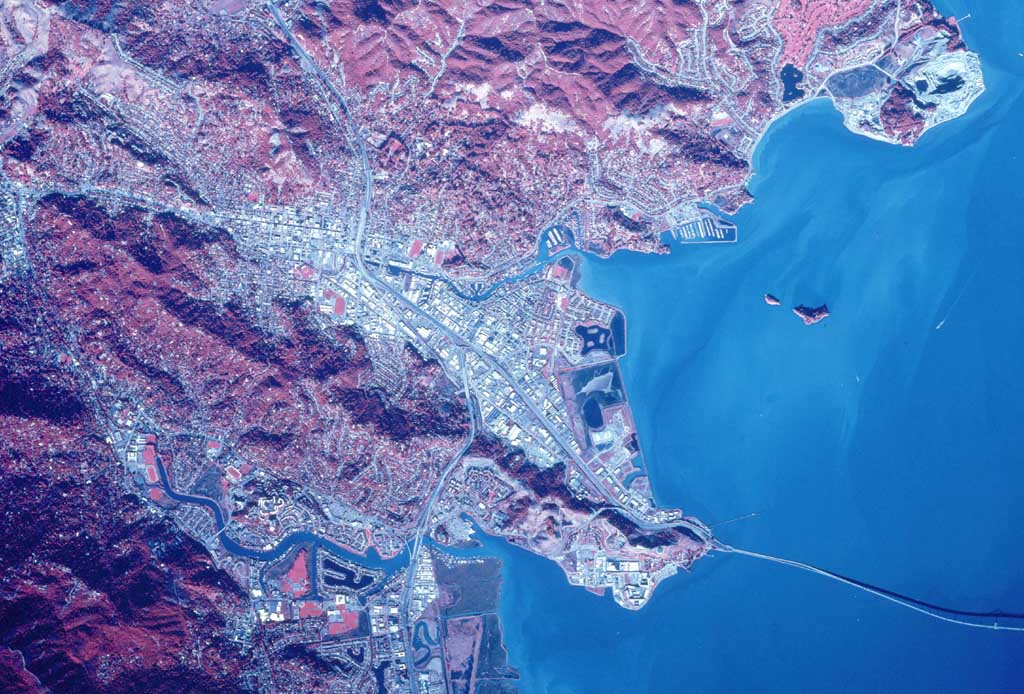This image showcases a stunning satellite view of a coastal region, marked with a striking red-like surface reminiscent of Mars. The left side of the image is dominated by a sprawling cityscape featuring a network of buildings and roads. This urban area is bisected by two rivers that flow gracefully toward the sea. 

The city extends onto a small peninsula that juts slightly into the ocean, which occupies the right half of the picture, depicted in serene shades of light and dark blue. The coastline features a combination of developed land and natural beauty, framed by sparse vegetation and mountainous terrain. A noticeable feature is a bridge extending from a middle peninsula into the ocean, suggesting developed infrastructure. 

In the ocean, two tiny islands are also visible—one slightly larger than the other. The settlement appears fairly compact yet developed, hinting at a remote location possibly designed for specific purposes. Additionally, a long road stretches from the city into the mountainous areas at the top of the image, connecting various parts of this unique landscape. This image offers a mesmerizing blend of natural and man-made elements, capturing the essence of a remote coastal development.